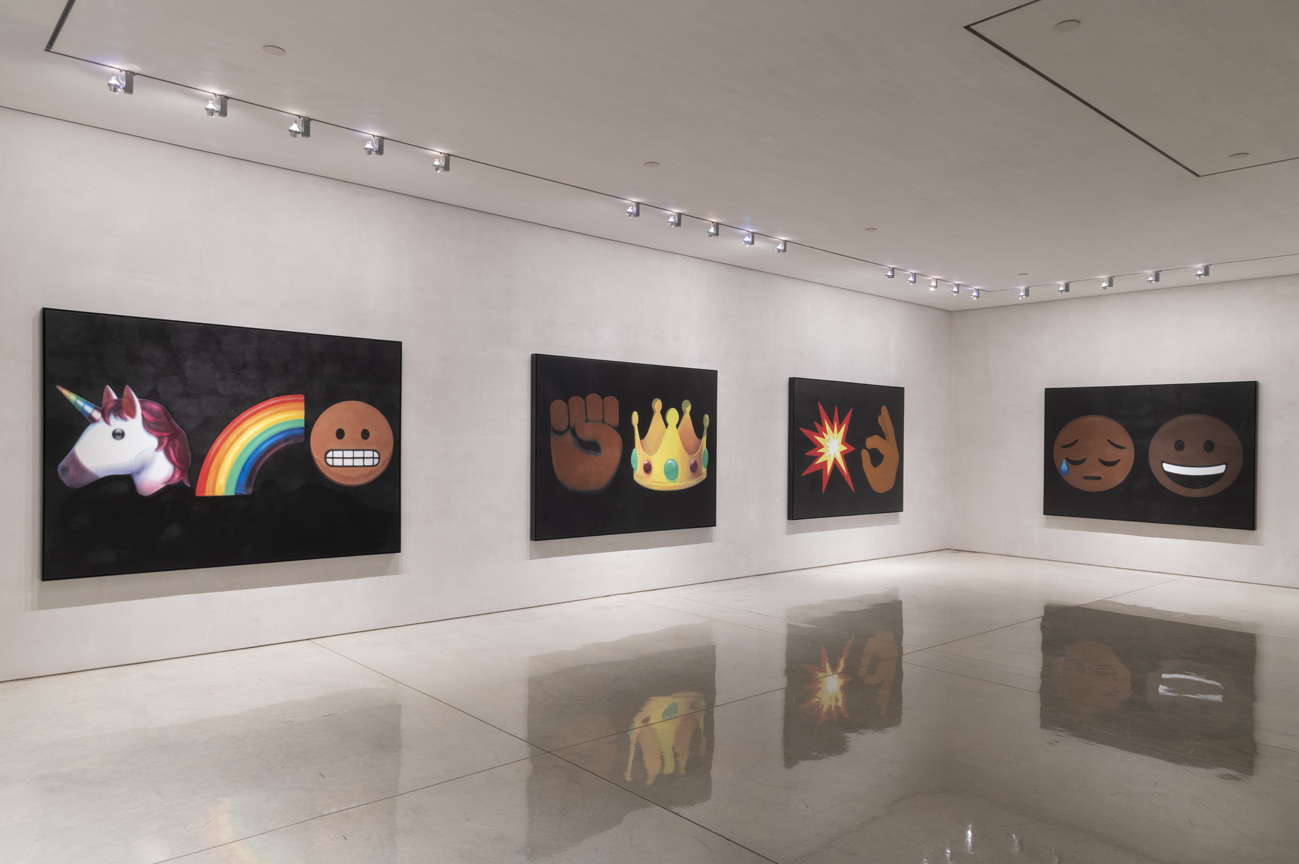The photograph, taken inside a modern art gallery, showcases a sleek and luminous space with glossy off-white marble floors accented by brown grout lines. The pristine white walls and ceiling, adorned with small track spotlights, elegantly illuminate four large black rectangular canvases. Each canvas prominently features vibrant, emoji-like art pieces that captivate the viewer with their dynamic use of color and emotion.

On the far left, the first canvas displays a fantastical white unicorn with reddish-purple hair, a multicolored rainbow horn, and a warm brown snout. Adjacent to the unicorn is a cheerful, brown-smiling emoji face with vividly bright rainbow hues gracing its background. 

Next to it, the second piece features a powerful juxtaposition: a proud brown fist symbolizing strength and solidarity is paired with a regal yellow crown embellished with turquoise and red gems, hinting at themes of empowerment and royalty.

The third artwork presents an intense scene with a hand, extending the forefinger and thumb in an 'OK' gesture, just beside a sparking flame that transitions from orange to yellow, evoking a sense of dynamic energy and light.

Finally, the last canvas on the right wall reveals a poignant narrative with two contrasting brown emojis. The left emoji, displaying closed eyes and a blue tear, conveys sadness, while the right emoji, with open eyes and a broad white-toothed smile, exudes happiness and optimism.

The meticulous lighting, the sparkling marble floor, and the minimalist white interior further elevate the dramatic and emotive quality of the art, creating an engaging experience for gallery visitors.